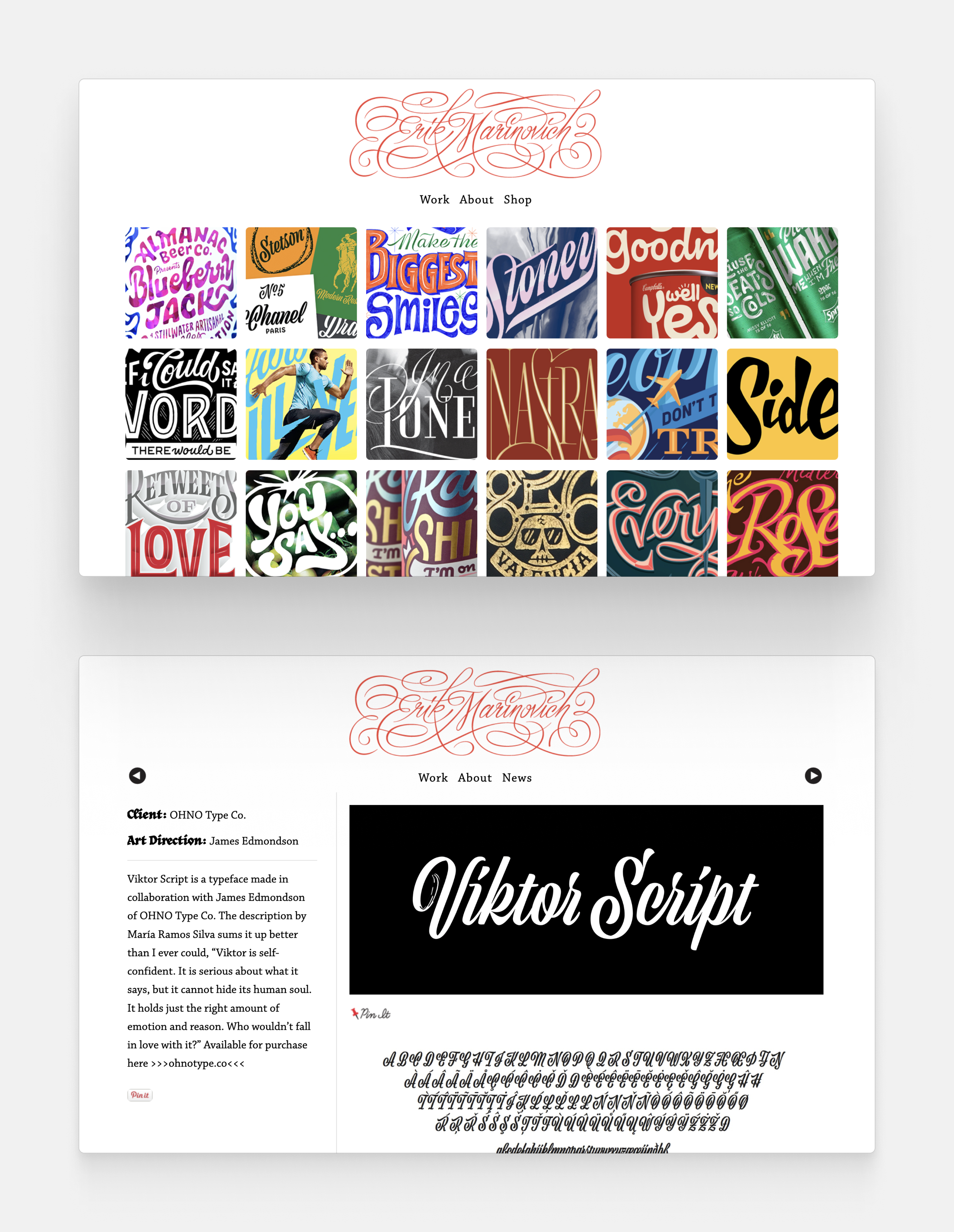The image showcases a web design mockup divided into two panels on a gray background, each framed in white boxes. The top panel features an elaborate, red, cursive logo that reads "VictorScript," surrounded by intricate curves, immediately drawing attention. Below the logo, simple navigation menus for "Work," "About," and "Shop" are present. This section displays a vibrant collage of 18 small images, each showcasing the VictorScript font in various colors and contexts—some appearing on labels, while others include words like "love," "side," and "rose," along with colorful everyday scenes in shades of purple, blue, green, gold, red, and more.

The bottom panel mirrors the top with the same cursive "VictorScript" signature. Below it, menus labeled "Work," "About," and "News" are visible. Dominating this section is a large black square with "VictorScript" written in bold white letters at its center. On the left side of this panel, there is information about the art direction and client, credited to James Edmondson. This bottom half seems to serve as a template for an "About" page, featuring further demonstrations of the VictorScript font design. The combined elements suggest this mockup is for a website showcasing the VictorScript font, highlighting its versatility and aesthetic appeal in a variety of design contexts.